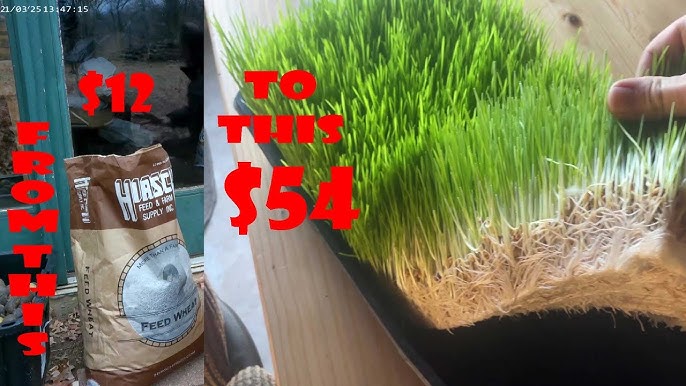The image consists of two side-by-side pictures forming an advertisement. The left picture features a brown sack labeled "High ASC Feed and Form Supply Ink" at the top, with a gray circle at the bottom displaying a picture of wheat and the text "Feed Wheat." Red text running down the side of this picture reads "From this," with "$12" prominently displayed above the sack. The right picture showcases a lush green lawn inside a black bucket, being held up at one end by a hand. Similar red text on this image states "To this," alongside "$54." The overall implication is that by using the feed wheat from the sack, one can grow valuable wheat grass, transforming a $12 investment into a $54 profit.